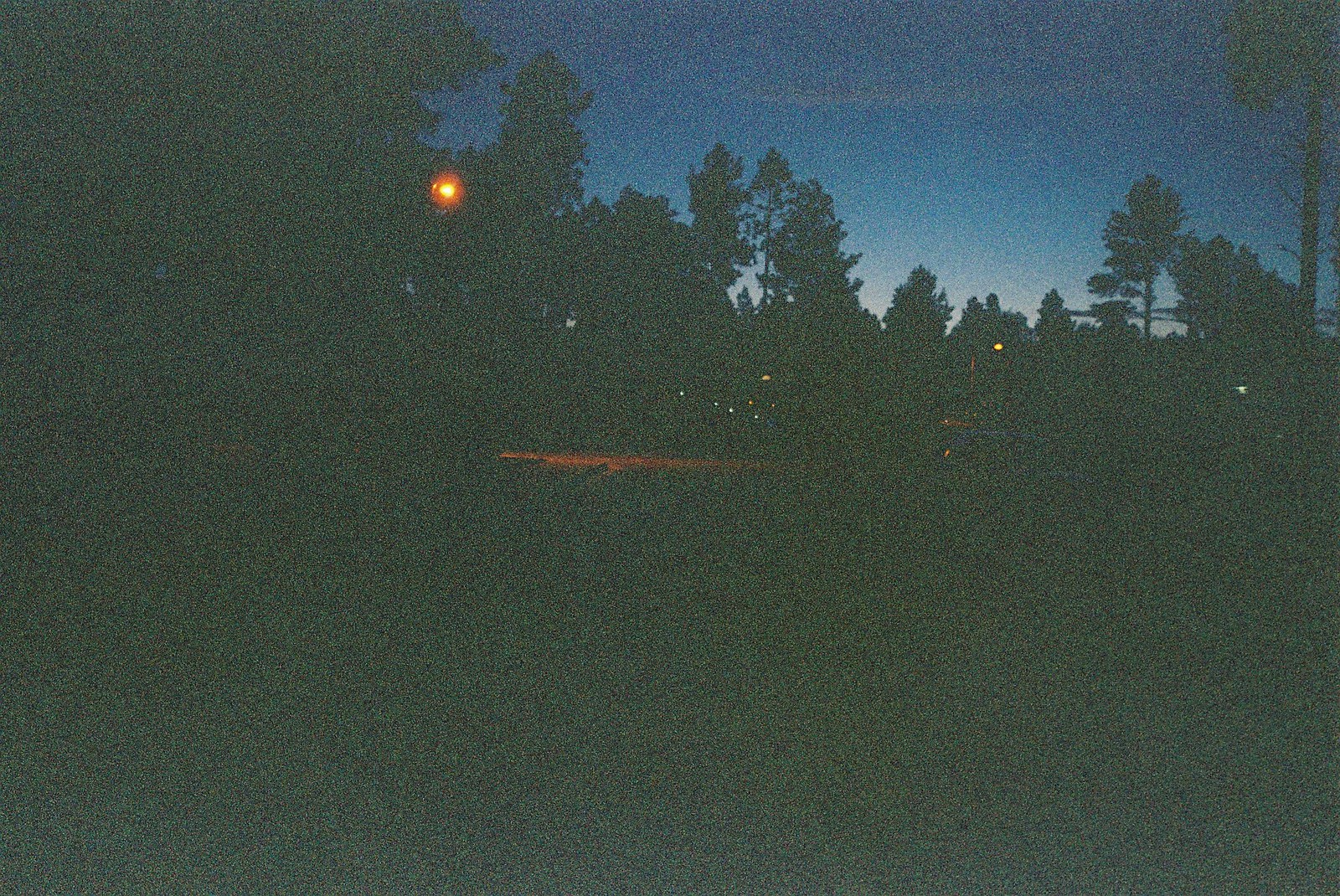This nighttime landscape photo captures the serene outlines of numerous trees in the background, softly illuminated by a lone streetlight in the top left corner. The streetlight emits a dim glow that barely penetrates the surrounding darkness, casting subtle highlights on the nearby trees. Despite the graininess of the image, you can discern the transitioning hues of the night sky, which shifts from a deep, dark blue at the top to progressively lighter shades of blue as it descends closer to the horizon.